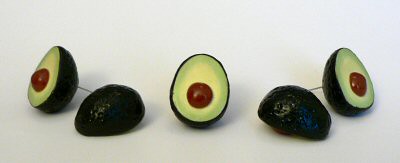This photo features five halved avocados meticulously arranged on an off-white background with subtle shadowing in the corners. At the center, a large avocado reveals its green flesh and chestnut-brown seed. Flanking this central avocado are two others, also sliced open to display their vibrant interiors and prominent pits. Between these three halves, the remaining two avocados are positioned cut-side down, showcasing their dark, textured green exteriors. The arrangement creates a pleasing symmetry, with each cut half paired with its counterpart facing down. The varied textures and colors—from the smooth, bright green flesh to the rugged, dark green skin—add depth and visual interest to the composition.